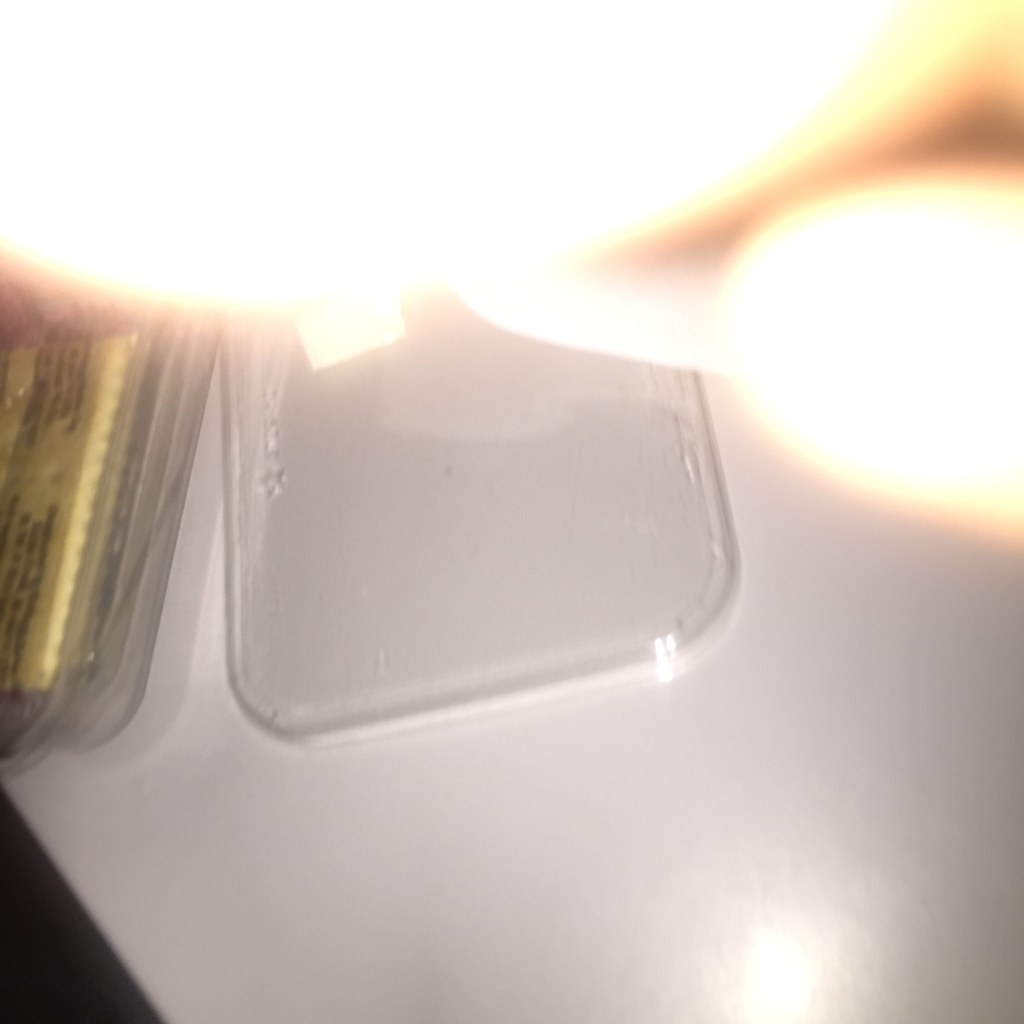A somewhat blurry photograph, capturing a scene with various elements. In the bottom left corner, a distinct black triangle can be seen. A white table occupies a significant portion of the image, its surface slightly obscured by a glaring reflection of sunlight near the bottom. On this table, there are two plastic containers; one appears empty, while the other contains crackers in a clear package adorned with black writing. The top portion of the image is dominated by an indistinct, large blur, featuring a blurry circle. To the right, there's a glowing, oval shape that resembles a fingerprint, adding an enigmatic touch to the composition.